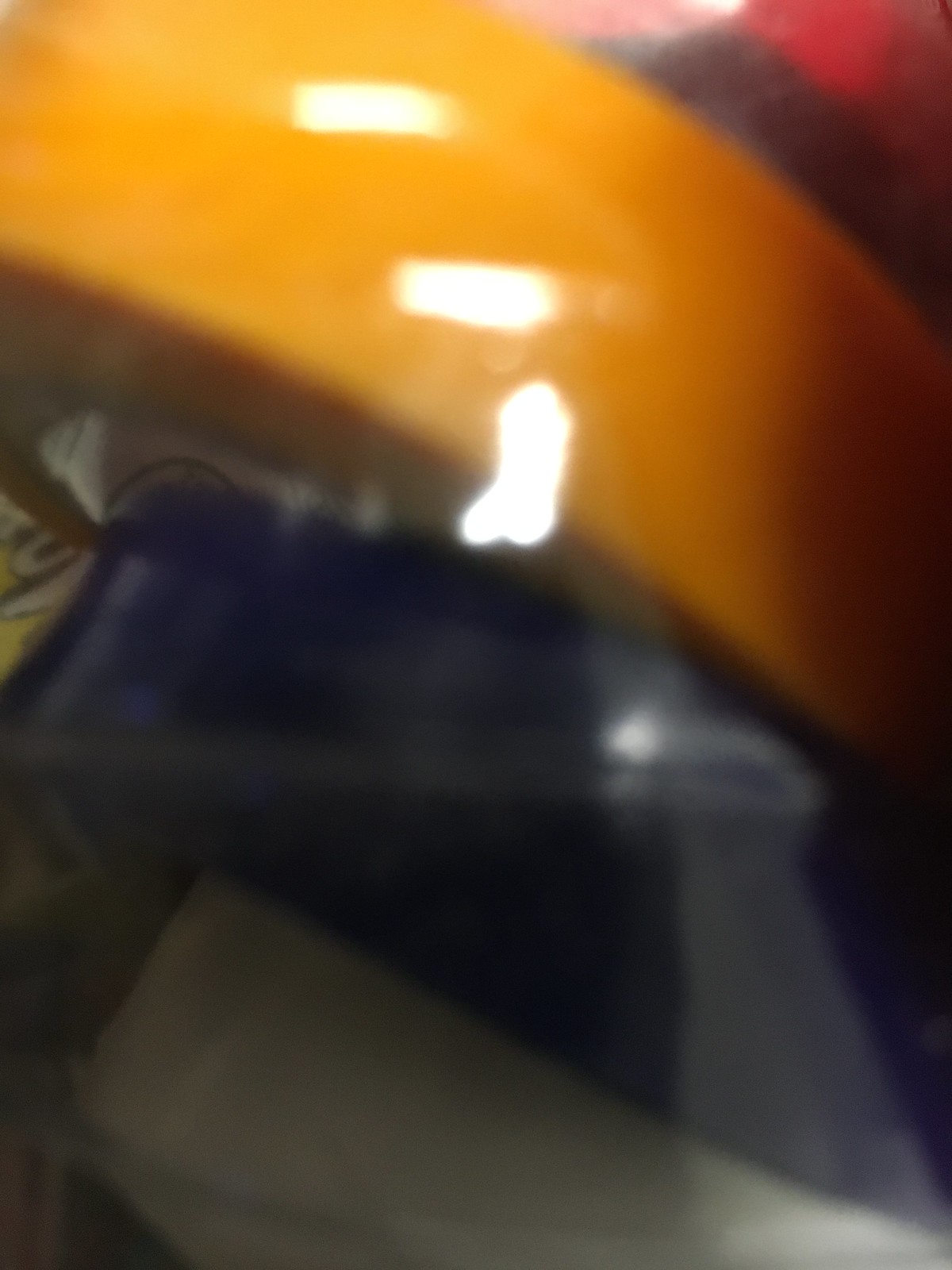In this extremely blurred image, there is a prominent yellow-orange circular object in the foreground, showing a curved edge that suggests it is mostly circular. The object is unusually shiny, almost resembling a large wheel of cheese but more reflective. Above this object, a blurred black line is partially visible, intertwined with a hint of pink. Above the black line, there is an indistinct red object that is too blurred to identify. The entire scene appears to be covered by some type of transparent plastic, with light reflecting off its surface. Below the yellow circular object, there is a blue item that also has a plastic-like appearance.